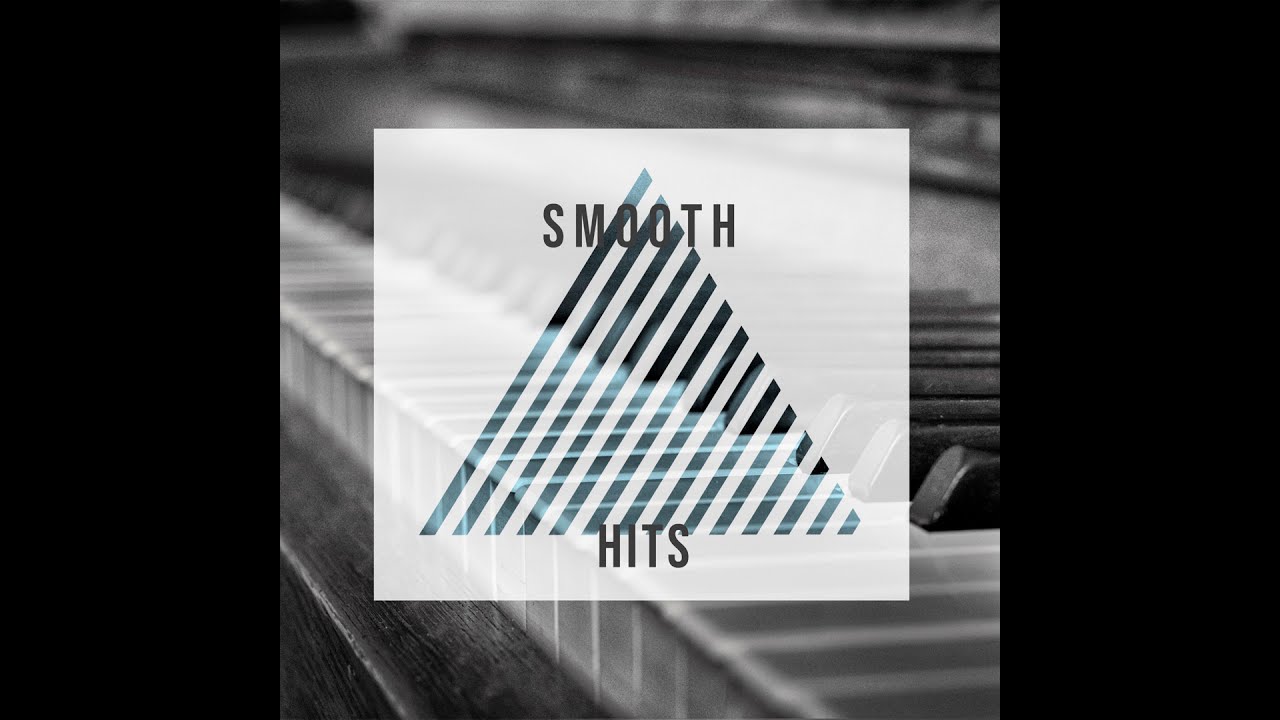The image displays a sophisticated black-and-white close-up of piano keys, captured at an askew angle where the nearer keys are in sharp focus, gradually blurring as they recede. Dominating the center foreground is a semi-transparent white square, within which sits a blue triangle composed of diagonal transparent stripes, allowing the piano keys to subtly show through. The piano is set against a backdrop that hints at rich, brown wood. The logo text, "SMOOTH HITS," is prominently overlaid on this triangle, with "SMOOTH" placed at the top and "HITS" at the bottom, both in capitalized gray letters. This image likely represents a logo for a music-related entity, perhaps a channel or podcast, elegantly fusing visual and musical elements.